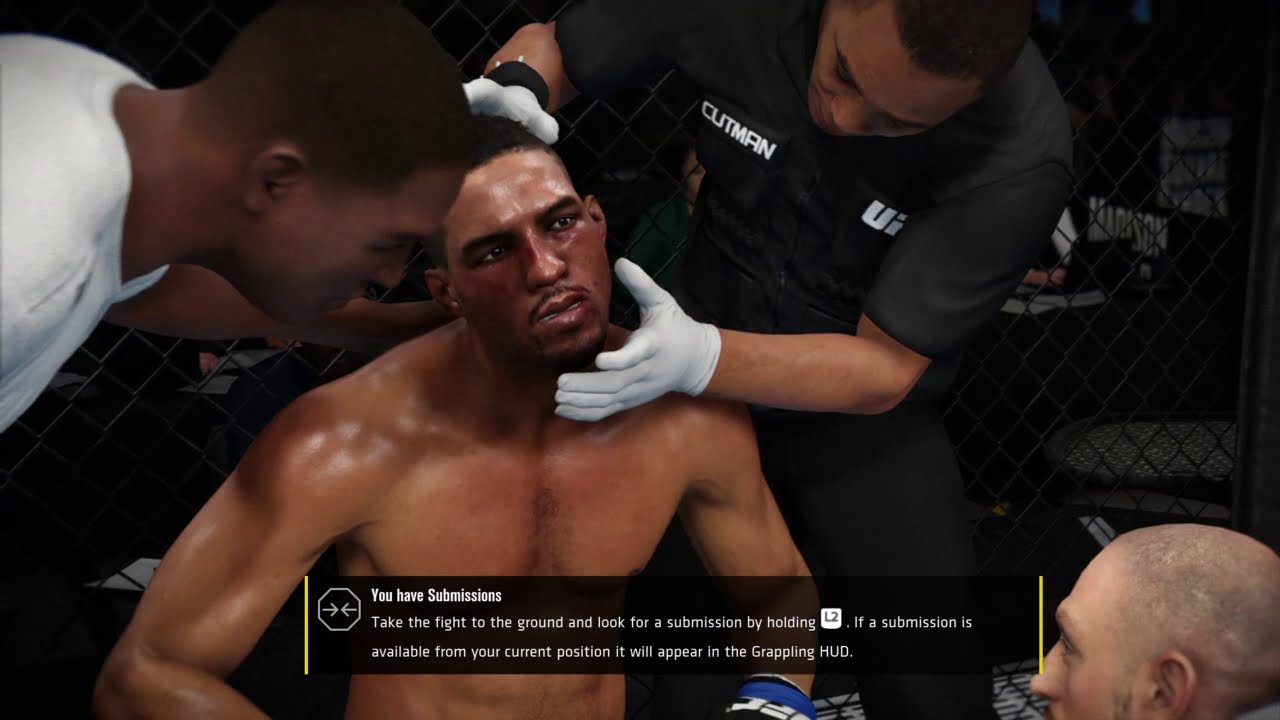The image depicts a highly realistic screenshot from a UFC fighting video game. It focuses on a muscular, shirtless African-American fighter seated in the corner of an MMA cage. He is visibly sweating and showing signs of facial injury, including redness around the nose and eyes, with a slight frown indicating discomfort. The fighter is wearing black and blue gloves, which likely bear the UFC logo. 

Two members of his support team are attending to him: one, an African-American man dressed in a black uniform with short sleeves and white medical gloves, is closely inspecting the fighter's face. The second team member, partly visible in the lower right-hand corner, is a bald Caucasian man, possibly the coach, who is attentively looking up at the fighter. Additionally, there is another individual in the upper left-hand corner, an African-American man in a white shirt, also focused on the fighter.

In the background, a chain-link fence typical of MMA cages is visible, suggesting the setting is within an arena. The bottom of the screen features a semi-transparent black box with white text providing gameplay instructions: "You have submissions. Take the fight to the ground and look for a submission by holding L2. If a submission is available from your current position, it will appear in the grappling HUD (heads-up display)." This annotation indicates that the viewer is indeed looking at a moment from a UFC-themed fighting video game.